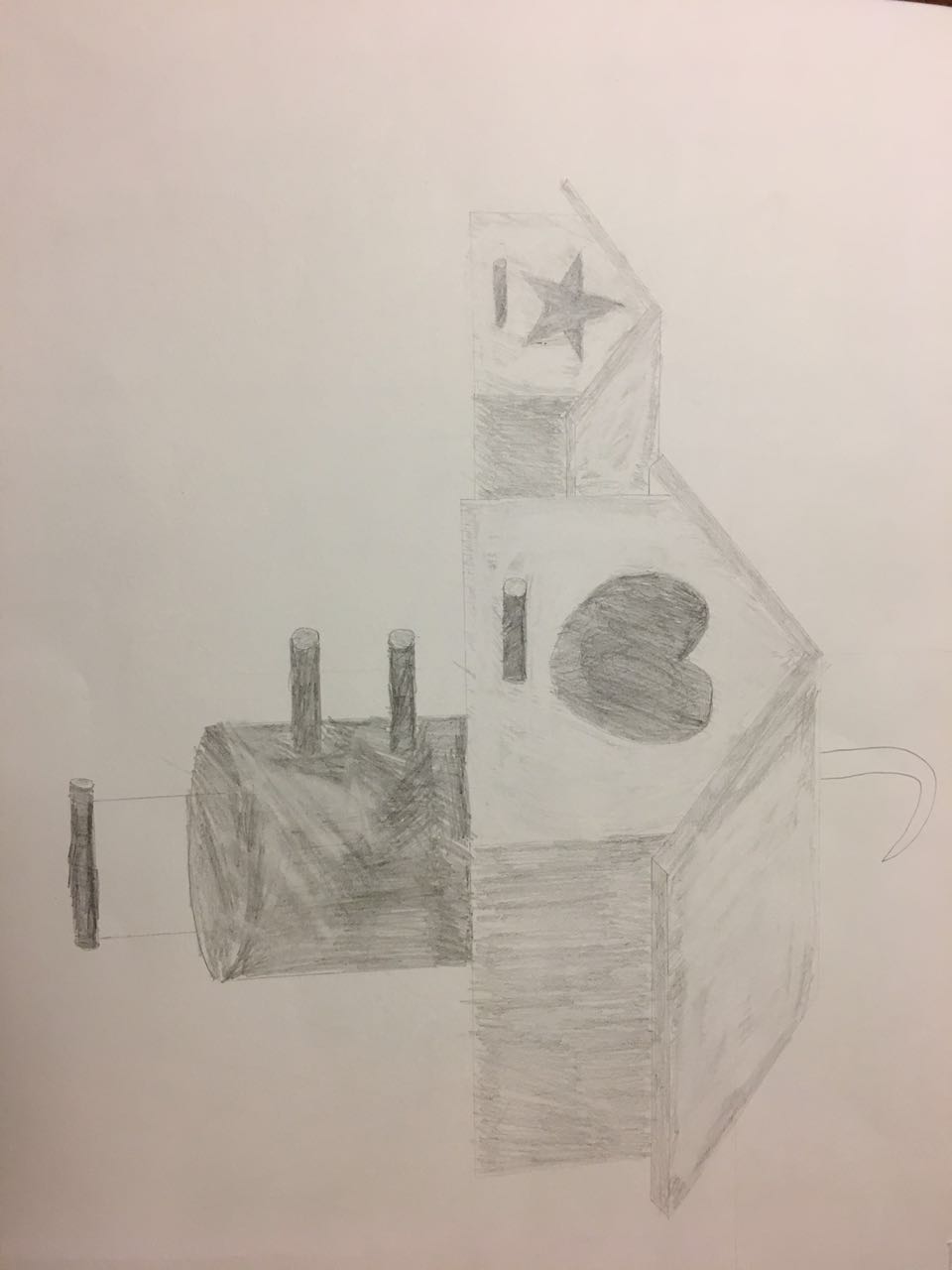This delicate pencil drawing, rendered in very light strokes, appears to be turned sideways. Set against an off-white background, it features a birdhouse with a slanted roof, crowned by a hook at the pinnacle. Centrally located on the birdhouse is a heart-shaped hole, framed by a short perch situated directly beneath it. Adjacent to this birdhouse stands a smaller variant, mirroring the design but with a star-shaped hole in place of the heart, complemented by its own perch.

Beneath these structures, a cylindrical form is depicted, incorporating two additional perches. Suspended below this cylinder is a swing-like element, complete with another perch at its base. The overall composition suggests a whimsical and inviting habitat for birds, meticulously illustrated in fine pencil lines.